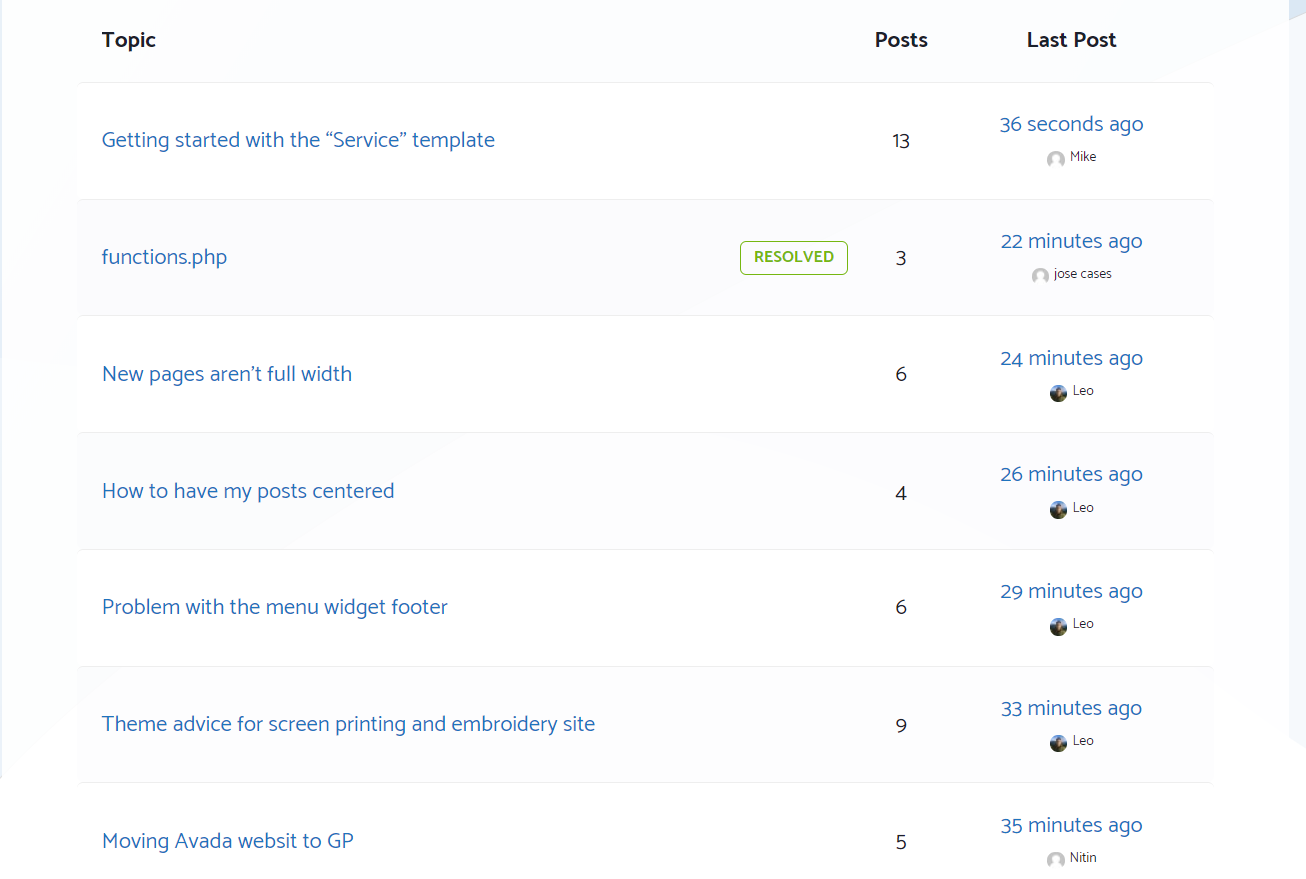Detailed description: 

The image depicts a screenshot of various forum threads presented in a tabular format. The table consists of three primary columns: "Topic," "Posts," and "Last Post." Each column neatly categorizes the information:

1. The first column, "Topic," lists the titles of the forum threads:
   - Getting Started with the Service Template
   - functions.php
   - New Pages Aren't Full Width
   - How to Have My Post Centered
   - Problem with the Menu Widget Footer
   - Theme Advice for Screen Printing and Embroidery Site
   - Moving a Vata Website to GP

2. The second column, "Posts," though not explicitly detailed in the provided text, would generally indicate the number of posts within each thread.

3. The third column, "Last Post," specifies how recently the latest post in each thread was made and by whom:
   - "Getting Started with the Service Template": Last post by Mike, 36 seconds ago
   - "functions.php": Last post by Jose Cases, shown as resolved with a green button on the right
   - "New Pages Aren't Full Width": Last post by Leo, time not specified
   - "How to Have My Post Centered": Last post by Leo, time not specified
   - "Problem with the Menu Widget Footer": Last post by Leo, time not specified
   - "Theme Advice for Screen Printing and Embroidery Site": Last post by Leo, time not specified
   - "Moving a Vata Website to GP": Last post by Nitin, 35 minutes ago

The forum threads are interactively designed, with the status of each thread (resolved or unresolved) indicated by a green button on the right side of the "Topic" column. Notably, only the "functions.php" thread is marked as resolved.

The textual elements of the table are primarily in blue, complementing the very light gray background of the screenshot. This color scheme provides a clear and aesthetic visual separation between the various elements of the interface.